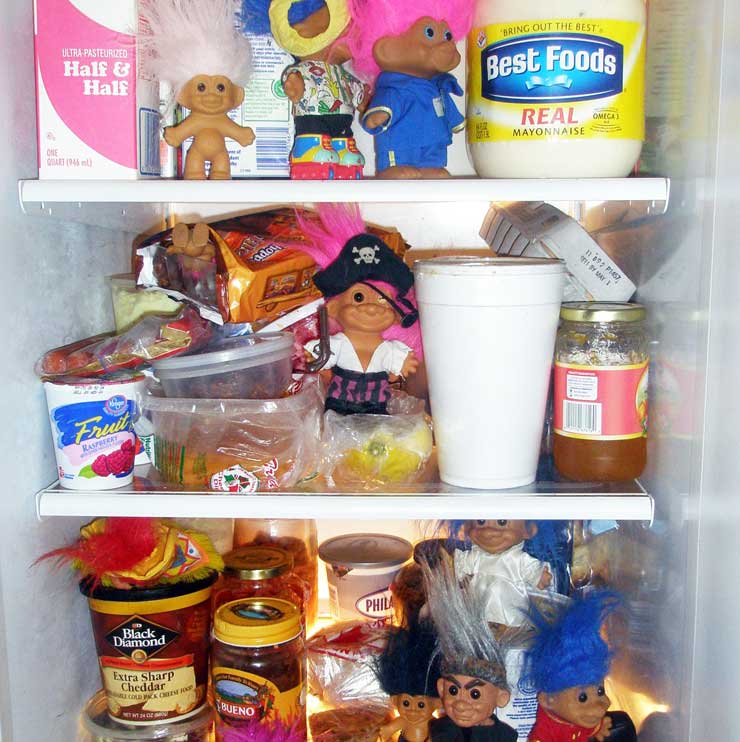The photograph captures the interior of a small, well-lit refrigerator with three white, glass shelves fully stocked with a variety of food items and an unusual assortment of troll dolls. On the top shelf, a carton of Half and Half sits next to some mayonnaise, with three troll dolls positioned between them—one with white hair, another with blue hair, and the third with pink hair. The middle shelf is cluttered with various food packages including a carton of eggs, a styrofoam takeaway cup, a jar of jelly, and a small yogurt container. Among these, a pirate troll with pink hair rests on a piece of fruit. The bottom shelf features items like Extra Sharp Cheddar, jars, and Philadelphia cream cheese. Here, four troll dolls reside on the right side—two with blue hair, one with gray hair, and one with black hair—while a red-haired troll doll lies on its belly on top of some Black Diamond almonds. The trolls, some dressed in outfits such as a pirate ensemble, and many in robes or without clothing, create a curious scene, suggesting either a whimsical artistic arrangement or an elaborate prank.